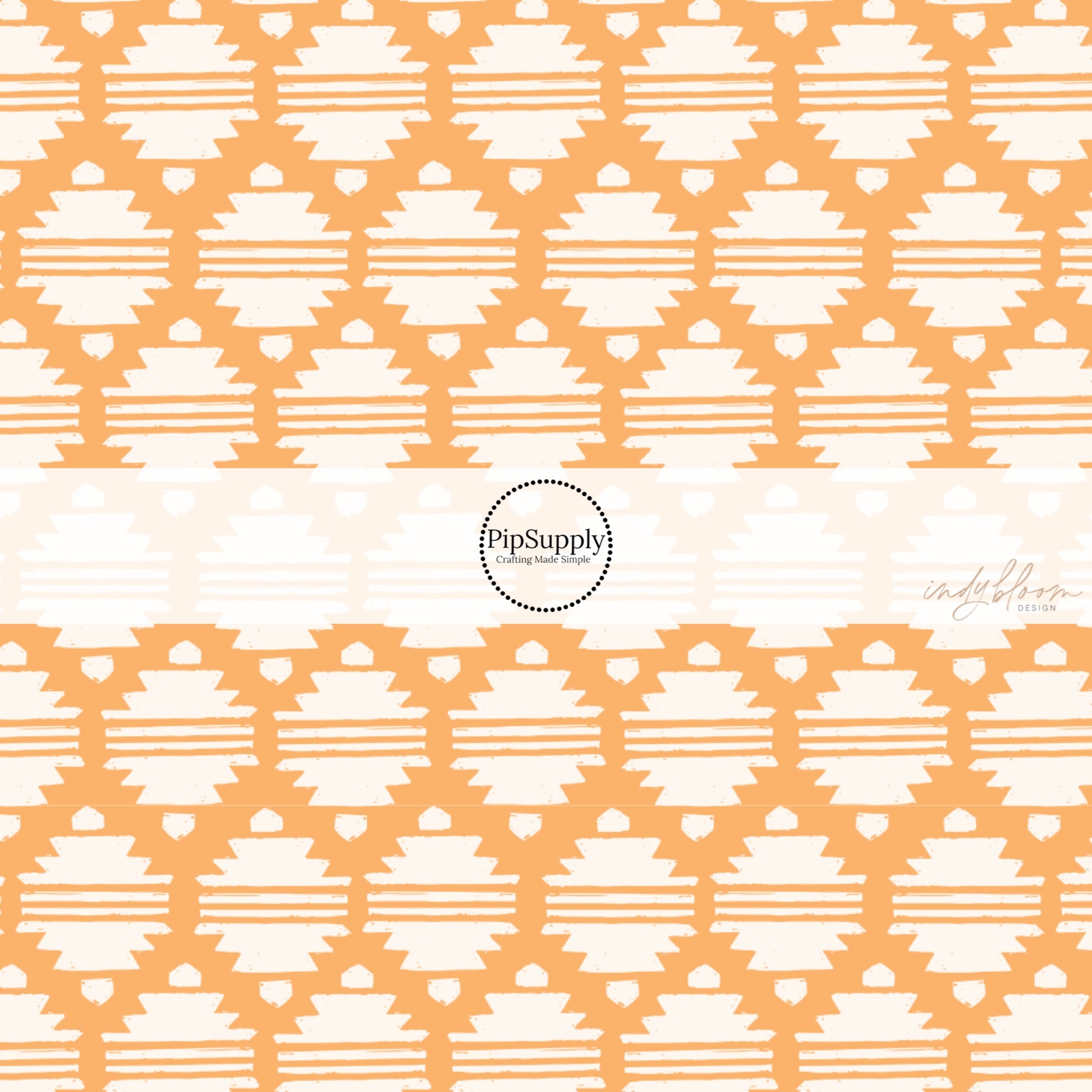The image appears to be the cover of a book or journal, predominantly featuring a peach shade of orange pattern against a cream-colored background. The design consists of geometric, diamond-shaped blocks connected by zigzag lines, with horizontal lines running across in sets of three, creating a repetitive and intricate motif. Dominating the center is a vertically placed white stripe, resembling a removable label. This stripe contains a black dotted circle surrounding the text "Pips Supply" and the tagline "Crafting Made Simple." To the right of this circle, in a cursive font, the name "Indie Bloom" appears, followed by the word "Design" in capital black letters. The orangish pattern at the top and bottom of the cover features alternating orange and white segments, enhancing the rhythmic and crafted feel of the overall design.